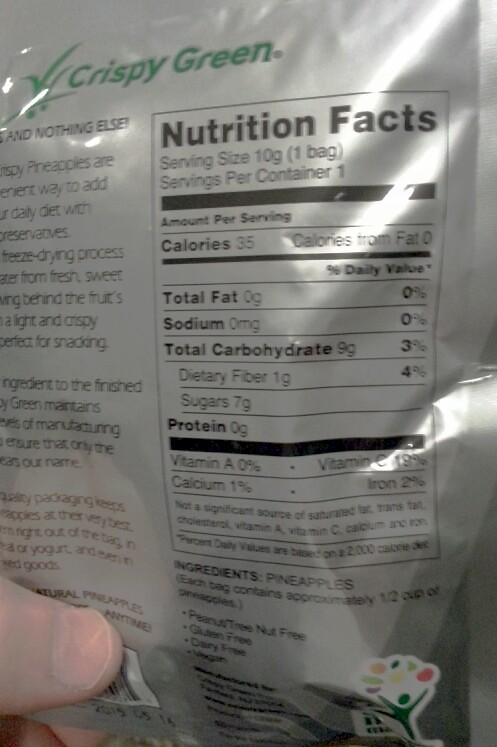The image shows a close-up of the back of a product package that is partially cut off on the left side. The package itself is silver-gray and has green accents at the top. The green section contains the brand name "Crispy Green" in bold letters. Below this, the nutritional facts are detailed in black text.

It lists the serving size as 10 grams, which equates to one bag, with one serving per container. The nutritional information is as follows:
- Calories: 35
- Calories from Fat: 0
- Total Fat: 0g
- Sodium: 0mg
- Total Carbohydrate: 9g (3% Daily Value)
- Dietary Fiber: 1g (4% Daily Value)
- Sugars: 7g
- Protein: 0g

The ingredients section mentions that the product contains pineapples, and each bag is approximately equivalent to half a cup of pineapples.

The image shows a person's thumb holding the package, obscuring part of the text on the right side. However, visible green text states that the pineapples undergo a freeze-drying process to preserve their sweetness, making them light and crispy—perfect for snacking.